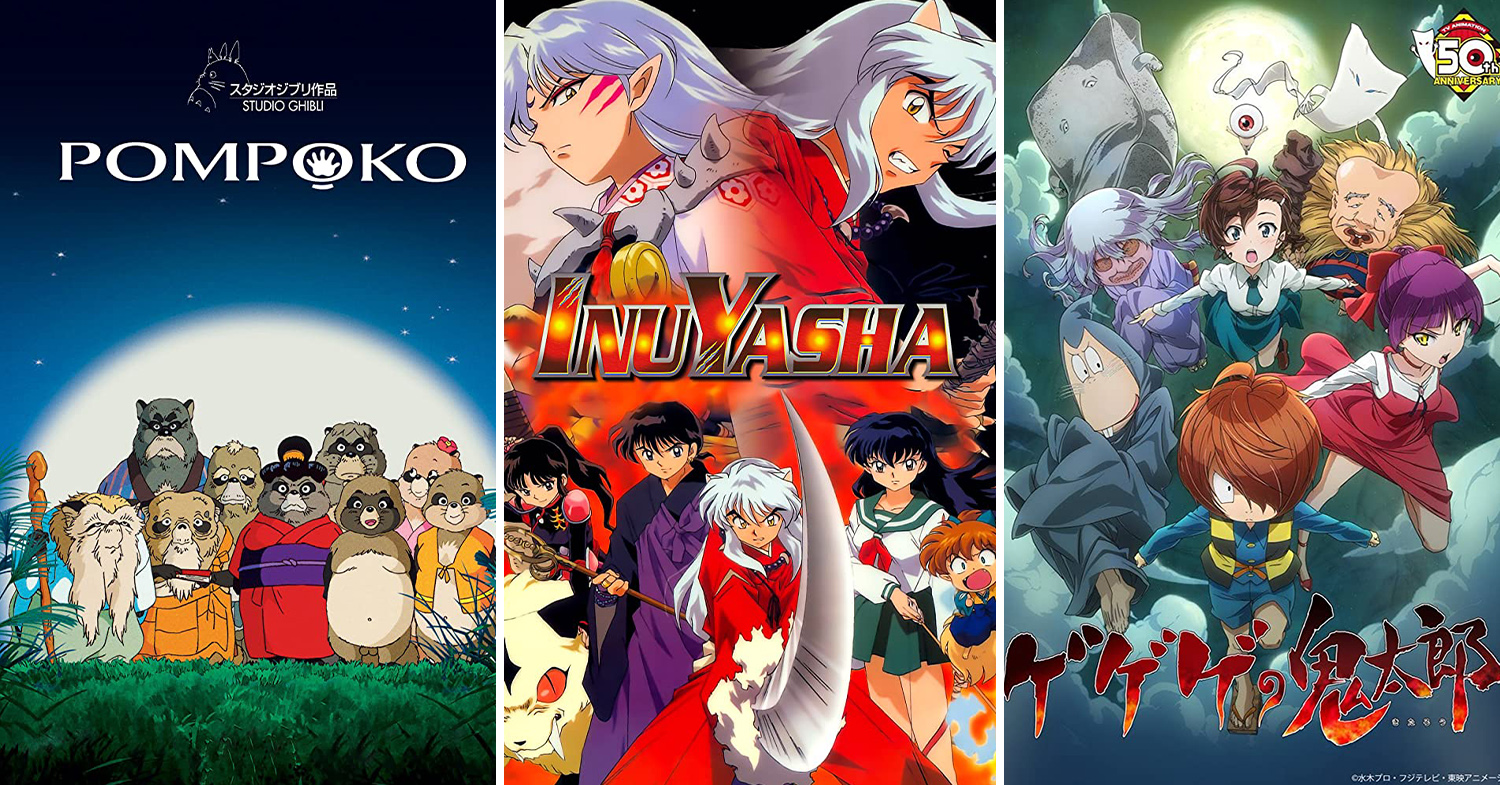The image showcases three distinct anime covers. On the far left is a cover for "Pom Poko" from Studio Ghibli, which features a nighttime scene with a prominent moon on the horizon. In the foreground, there is a family of anthropomorphic raccoons and other animals, all clothed and smiling, standing on a grassy field under a starry sky. The middle cover is for "Inuyasha." It prominently displays a character in a red robe wielding a sword, likely Inuyasha himself, with additional characters around him, including a figure in a purple robe that might be a magician. The characters exhibit a mix of white and black hair, some with pointed elf-like ears and carrying weapons, set against a dynamic and colorful background. The cover on the right, although the title is in Japanese and not clearly identifiable, features a group of various characters with distinctive appearances, including a girl with purple hair in a red dress, set against a nighttime backdrop with a moon. The characters are shown in action poses, possibly jumping or engaging in some activity, surrounded by a myriad of colors like black, white, gray, green, brown, blue, yellow, purple, orange, and red.